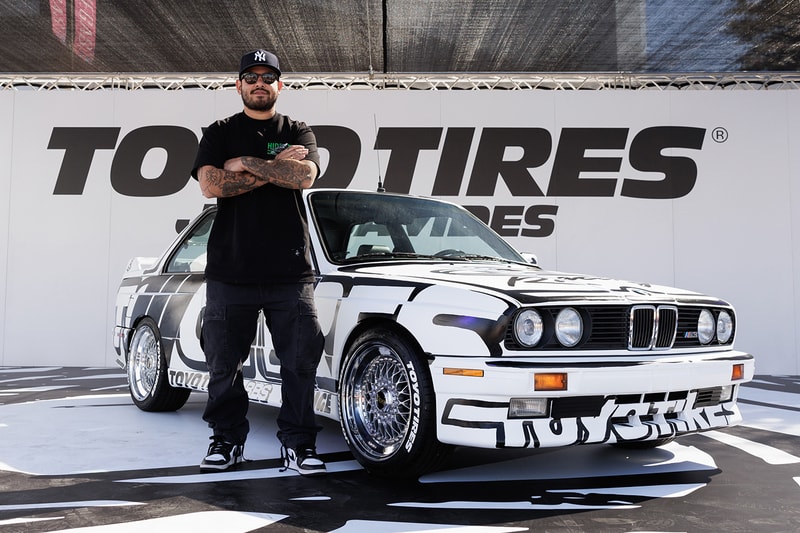In this detailed photograph, a young Hispanic man is posing confidently with his arms crossed in front of a customized sports car. The man is dressed in a black outfit, including a New York Yankees cap, sunglasses, a black t-shirt, black pants, and white and black Nike sneakers. His forearms are fully tattooed, adding to his distinctive look.

Behind him is a large banner advertisement for "Toyo Tires," partially obscured by the man's position. The background also includes additional obscured text and a logo on the tarmac, suggesting a promotional setting or a raceway. 

The car itself is strikingly customized with a black and white paint job and prominently features Toyo tires. It boasts four headlights and stylish rims, and while the front grille shows a BMW hood, it includes an unfamiliar logo with a number three on it. The car, angled to the left, showcases its unique design and craftsmanship, making the scene visually dynamic.